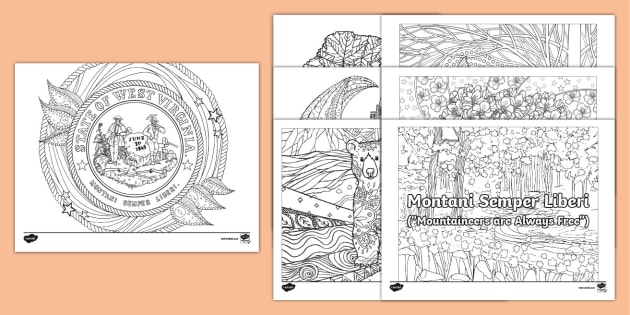This image features two side-by-side black and white illustrations on white paper against a peach-colored background. On the left side, there is an outline styled like a coloring page, depicting the state seal of West Virginia. The seal is round and contains the text "State of West Virginia" at the top and a partially obscured Latin motto that appears to include the word "Libri." Central to the seal are two figures—one wearing a large-brimmed hat and the other with a pickaxe—standing beside a rock inscribed with the date "June 20, 1863," marking the state's founding date. Surrounding the figures are rudimentary line drawings of trees, a wreath of leaves, and stars.

On the right side, there are six overlapping printer pages, each featuring different scenes emblematic of West Virginia. These include a forest scene with a creek and flowers, a bear, various floral illustrations, and other images of plant life. Overlaid on these illustrations is the Latin phrase "Montani Semper Liberi," which translates to "Mountaineers are always free." The thick black lines of the images suggest they are designed for coloring, making them ideal for educational purposes, such as teaching children about West Virginia's natural and historical heritage.